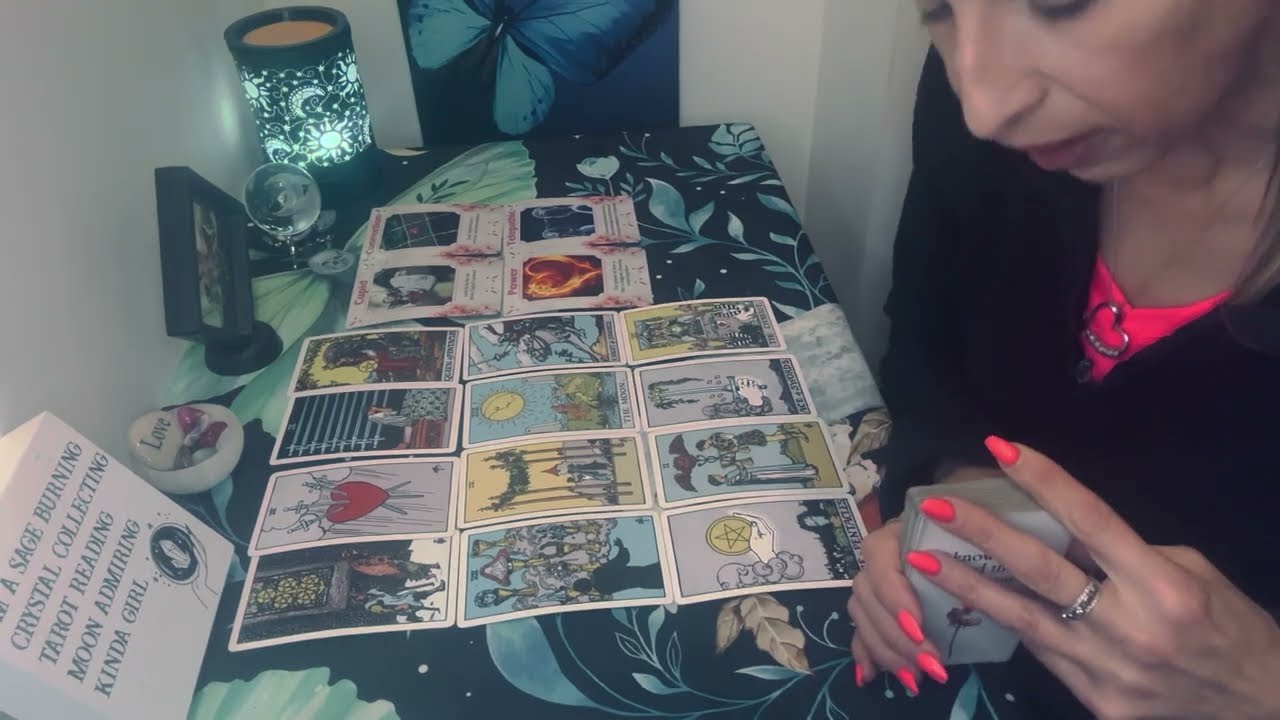The image captures a woman engaged in a tarot card reading session at a small, rectangular table adorned with a dark, floral-patterned tablecloth. She is arranging her tarot cards in three rows of four, with an additional set of four lighter-colored cards at the end. The woman, who is wearing a bright fluorescent pink shirt and a heart pendant necklace, has a black button-down sweater layered over her shirt. She has applied matching bright pink nail polish and has a ring on her middle finger. In her hands, she holds a stack of tarot cards. The scene is set within a room with white walls, which features a plaque on the table with the words "I'm a sage-burning, crystal-collecting, tarot-reading, moon-admiring kind of girl," and a rock inscribed with the word "love." A candle is lit nearby, and a fairy lamp and a poster of a blue butterfly can be seen in the background.